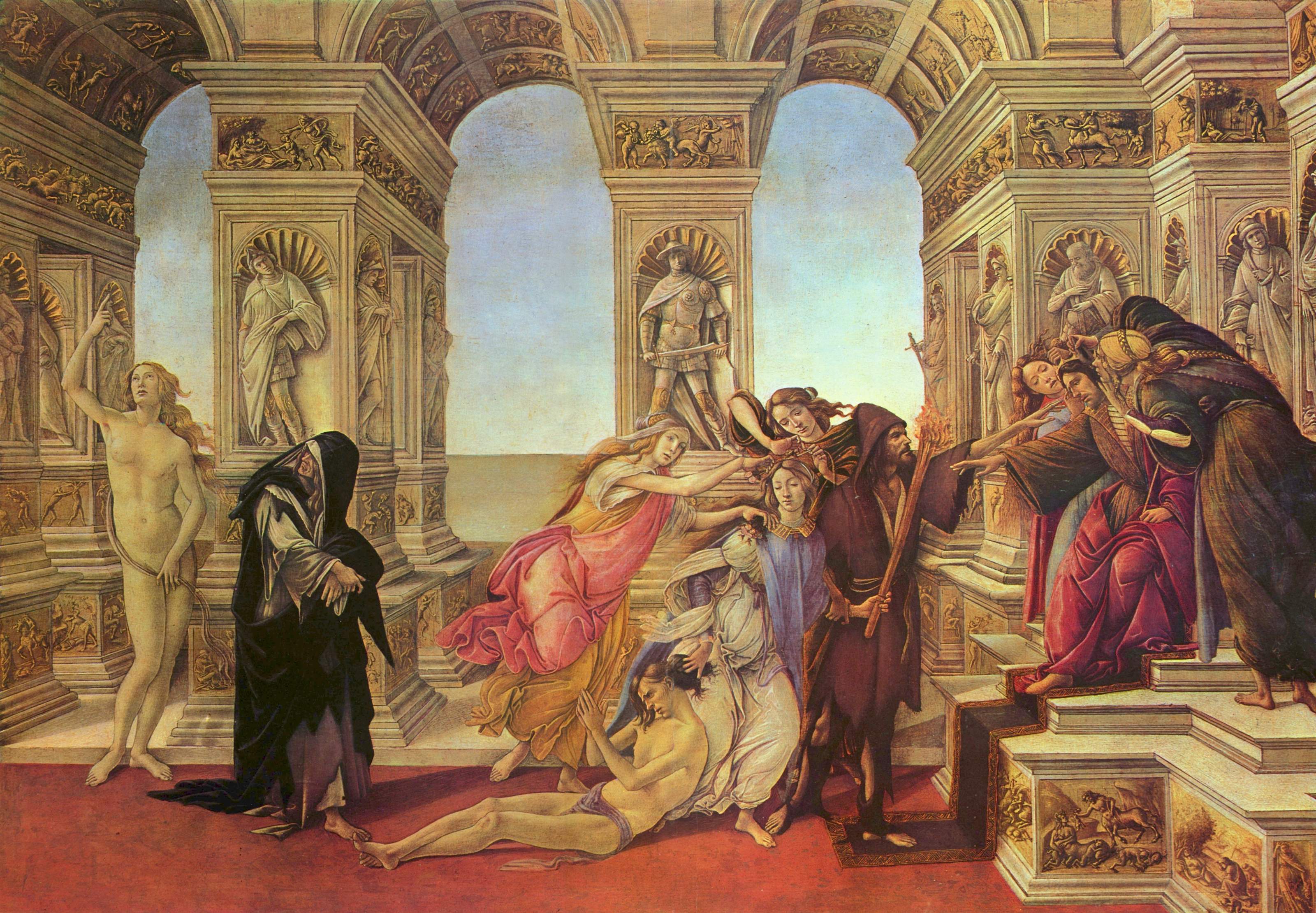The detailed painting appears to be set in an opulent throne room featuring Roman or Greek architectural elements, such as arches and pillars adorned with statues of figures in armor and robes. The central focus is a man, possibly a king, seated on a raised white stone platform. Beside him are two individuals gazing intently at him. In front of the king, a man in a tattered purple robe extends his arm towards the throne. Surrounding them is a small crowd, including a nearly naked man on the ground wearing only a loincloth. Another nearly naked man stands with long hair, his left arm covering his genitals and his other arm pointing upwards. The background shows arched windows overlooking a blue sky with clouds. Among the figures are women in various dresses, one in pink and brown with reddish hair, and another in blue and white, also with reddish hair. A cloaked man in black and a witch-like character add to the diverse assembly. The floor is a striking red, enhancing the grandeur of the scene.